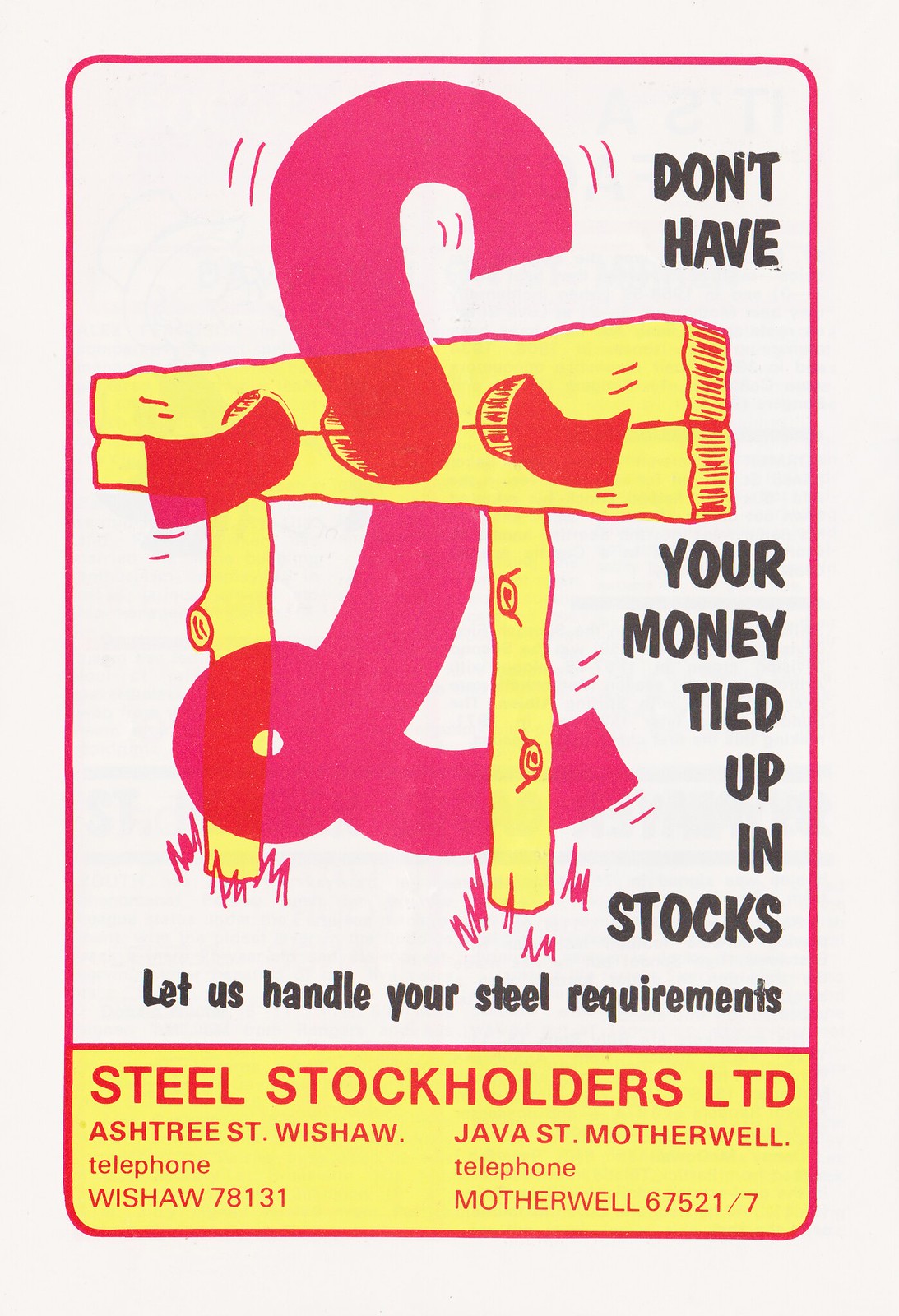This image is a vertically aligned rectangular advertisement for Steel Stockholders Limited, featuring a retro design with bright colors. It has a very light gray background with a vertical rectangular area outlined in dark pink. Inside this area is a large, curved, pink letter resembling a capital 'L' or an 'at' sign, intersected by two wood posts with a wood crossbeam. Black, right-aligned, capitalized text on the right side reads, "DON'T HAVE YOUR MONEY TIED UP IN STOCKS." Centered at the bottom in black letters, it says, "LET US HANDLE YOUR STEEL REQUIREMENTS." Below this text, there's a separate section with a yellow background and red text stating, "STEEL STOCKHOLDERS LIMITED." This section also includes contact information: "ASHTREE ST WISHAW TELEPHONE: WISHAW 78131" and "JAVA ST MOTHERWELL TELEPHONE: MOTHERWELL 67521/7."